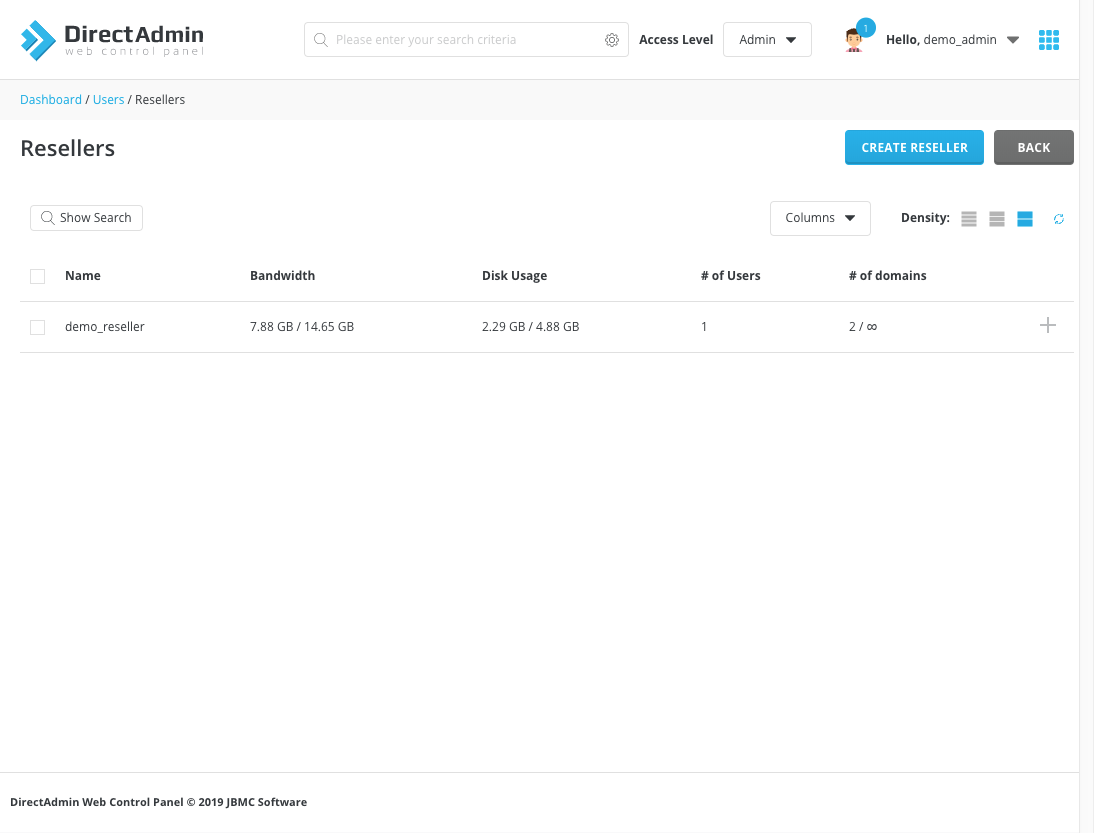The image is a screenshot of the Direct Admin Web Control Panel website, featuring a predominantly white interface with a rectangular layout that is slightly wider than it is tall. In the upper left-hand corner, there is a double blue caret logo followed by the text "Direct Admin Web Control Panel." The user is logged in as "demo_admin" and has one notification.

The current page is nested under the path "dashboard/users/resellers," which is indicated in a gray rectangle. The navigation labels "Dashboard" and "Users" are highlighted in blue, while "Resellers" is specifically focused on and lists "demo_reseller" as the sole entry. The resource metrics for the reseller include a bandwidth usage of 7.88 GB out of 14.65 GB and a disk usage of 229 GB out of 488 GB. Additionally, it indicates there is one user and two domains associated, with the number 2 followed by an infinity sign, suggesting unlimited domains.

At the top of the page are two prominent buttons: a blue "Create Reseller" button and a gray "Back" button. This page serves as an administrative control interface, offering detailed management capabilities for resellers within the Direct Admin platform.